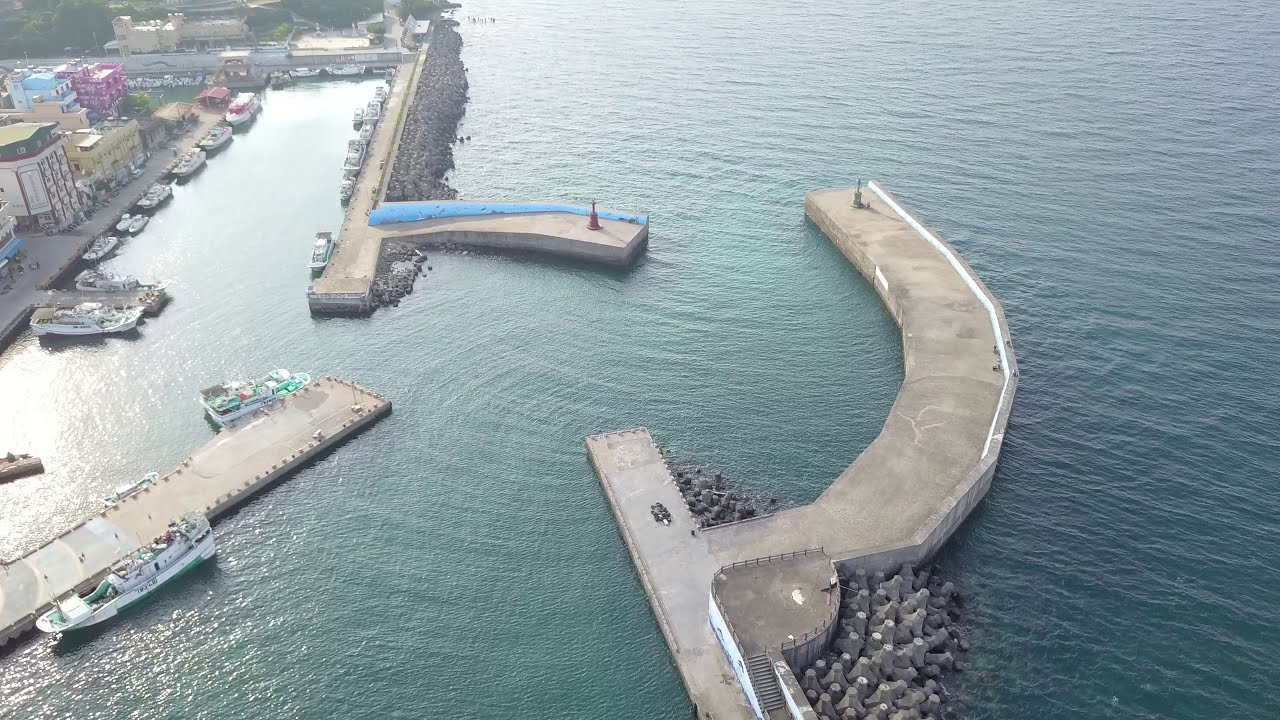This aerial photograph, captured on a bright sunny day, offers a stunning view of a marina nestled within calm, deep aquamarine waters. The landscape-oriented image reveals the marina's intricate layout, featuring multiple man-made structures and docks. Prominently, a curved jetty extends from the center towards the right, complemented by another jetty emerging from the left, beside which a boat is docked. Further enhancement comes from a rocky breakwater on the opposite side, ensuring the marina's protection. In the top left corner, a collection of boats are moored along a cemented edge, adjacent to a vibrant cluster of colorful buildings—pink, yellow, and blue—indicative of residential or commercial spaces. Tiny figures of people are visible, adding life to the scene. Overall, this detailed representation encapsulates the serene and bustling nature of the marina, framed by the penetrating blue of the ocean.